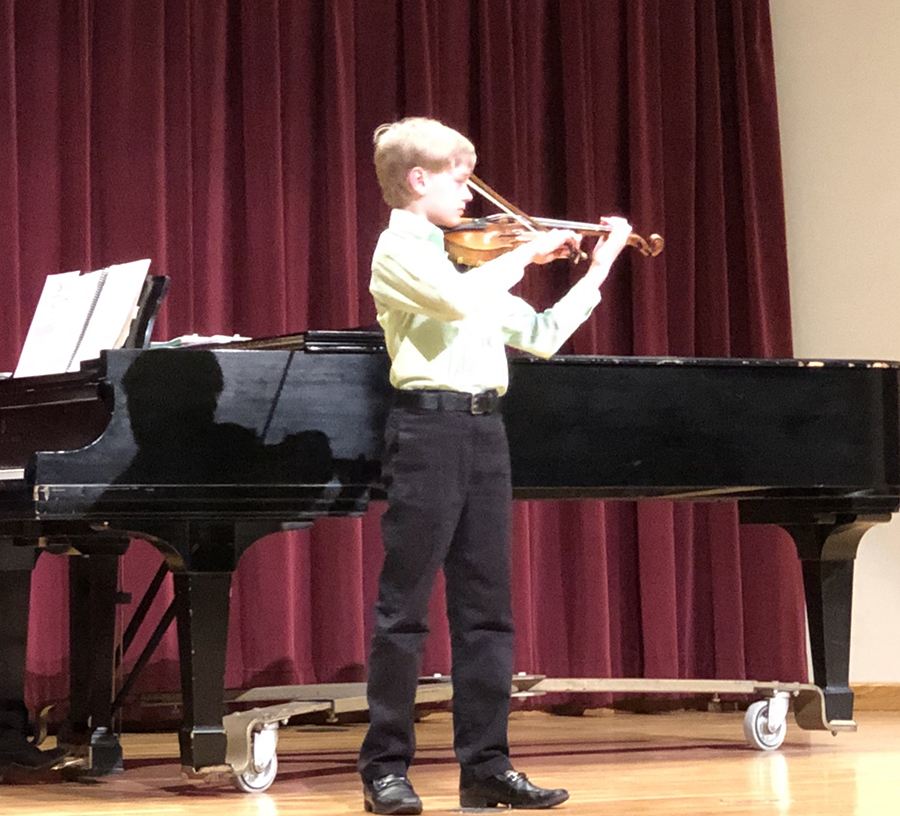In this detailed image, a young boy is the focal point, standing center stage on a light brown, wooden floor. He is performing passionately with a brown wooden violin in his hands. The boy is dressed smartly in a light green or white button-up shirt paired with black pants, a black belt, and shiny black dress shoes. Directly behind him sits a large black grand piano on a brown base with casters for easy movement and an open book resting on its top. The scene is framed by a plush, burgundy velvet curtain that covers most of the background, adding a sense of elegance to the setting. To the right of the curtain is a beige or yellow wall. The overall setting appears to be a school concert or recital, possibly an intimate moment captured by a proud parent. The image is devoid of any text, allowing the viewer to focus entirely on the young musician and his surroundings.